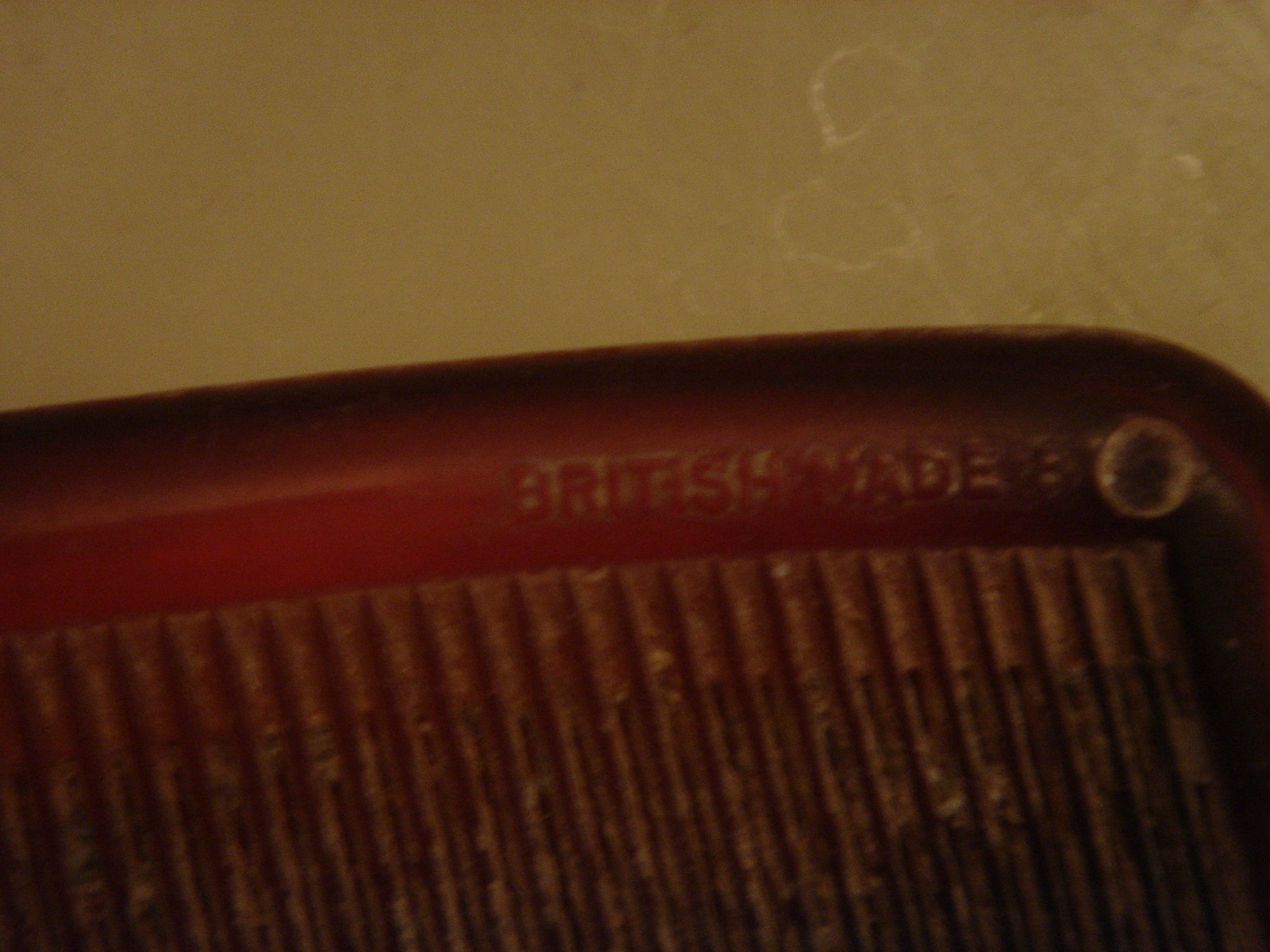The image depicts the top right corner of a mysterious object that appears to have a segmented design. The object, possibly a comb or a grill, is a dark maroon color that suggests it might be made of plastic, though this is not certain. Engraved on the long, red tubular edge of the item are the words "British made," though the text following this is not legible. The object is resting on a surface that is a mix of white and off-white with a hint of yellow. 

A notable feature of the object is a small circular element at one end, which could indicate that it is designed to be mounted or placed on a surface. Below the circular element, there is a pattern that resembles a wasp nest, composed of multiple small tubes aligned next to each other, each with faint black lines running through them. This intricate pattern enhances the resemblance to a grill, though its true function remains uncertain.